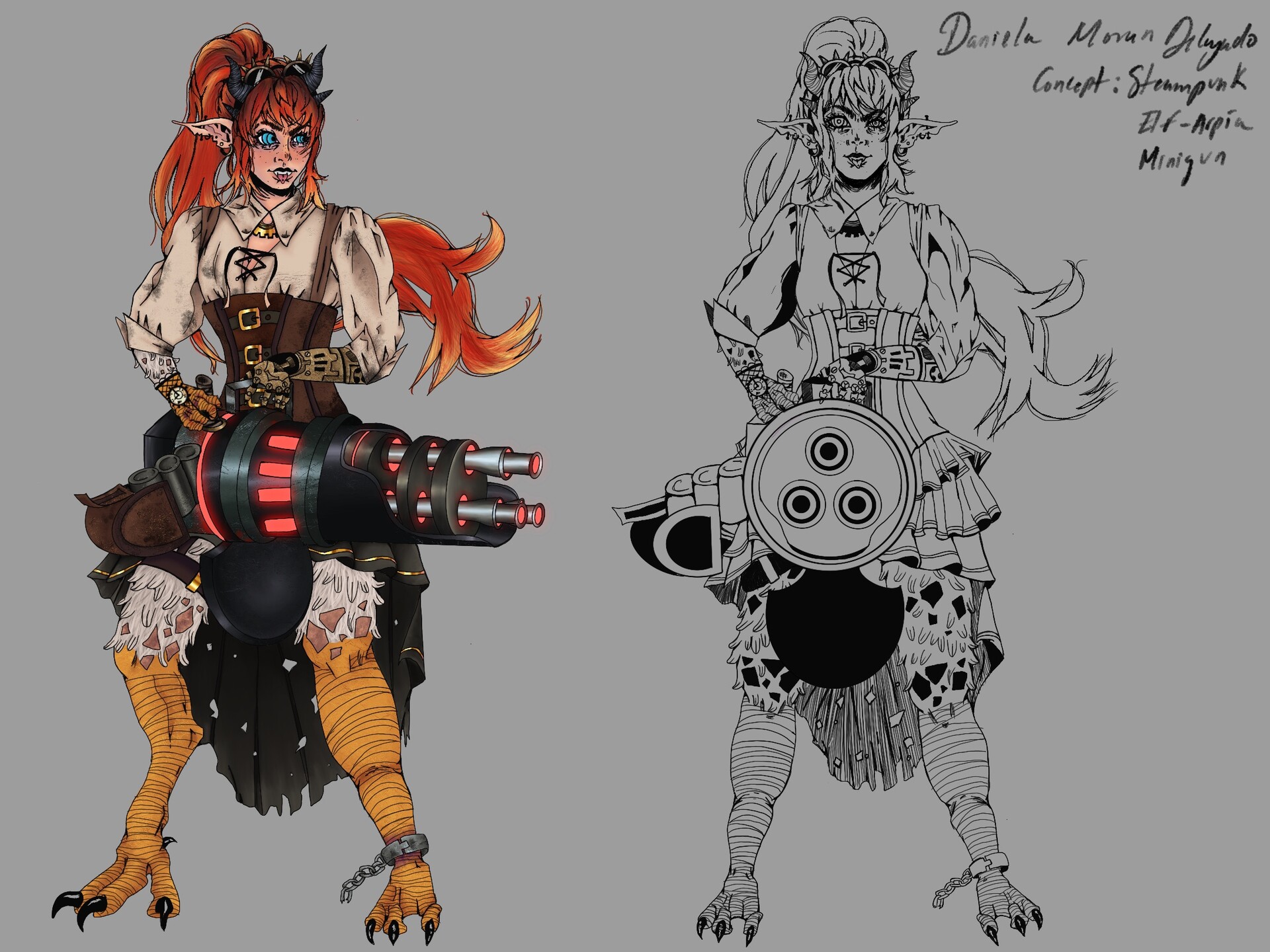The image features a detailed, colored sketch of a female character with a distinct steampunk aesthetic. She has long red (or orange) hair and large, pointed ears. One hand appears robotic while the other is ambiguous, possibly metal or bird-like. Her attire consists of a beige peasant blouse with puffy long sleeves, laced in the front, and a brown dress featuring buckles and an uneven hemline that extends to her knees in front and down to her ankles in the back. She also has a chain around her left ankle. Her legs have a bird-like quality, with webbed feet and claws, resembling those of a bird, and are wrapped in bandages up to where the dress begins. She is holding a large, black weapon with red accents, possibly a laser gun or machine gun. Next to the colored drawing is a black and white sketch of the same character, highlighting her weapon from a frontal view. In the top right corner of the artwork, the text reads, "Daniella Morin. Concept, Steampunk, Elf, Arpeia."